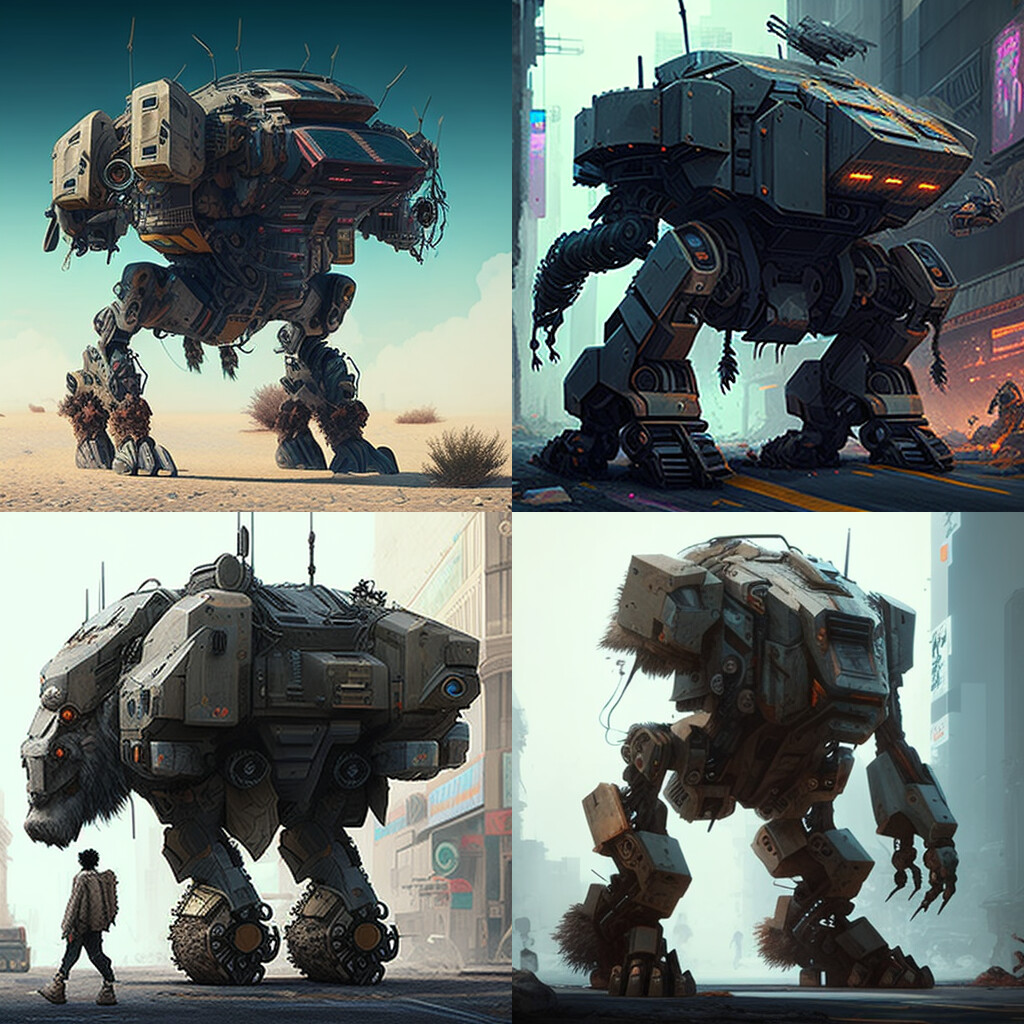The image is a composite of four distinctive illustrations of Battletech-type mechs, each occupying a quadrant of the picture. In the bottom left, a hybrid creature combines both organic and robotic features, with a noticeable face and furry tufts around its body, suggesting a fusion of flesh and metal. A human figure walking beside it highlights the mech's imposing size. The bottom right mech, despite having only one arm, also displays organic attributes with fur protruding from its feet, back, and amputated arm area. The mech in the upper right embodies a classic bipedal Robotech tank, armed with potential weaponry on its top, though it's slightly obscured by what might be background effects. The upper left mech, stationed in a desert landscape, resembles a bison with four fur-adorned legs and barely discernible eyes, blending natural and mechanical aesthetics. Each mech appears battle-worn and aged, further enhancing their intricate and detailed designs.